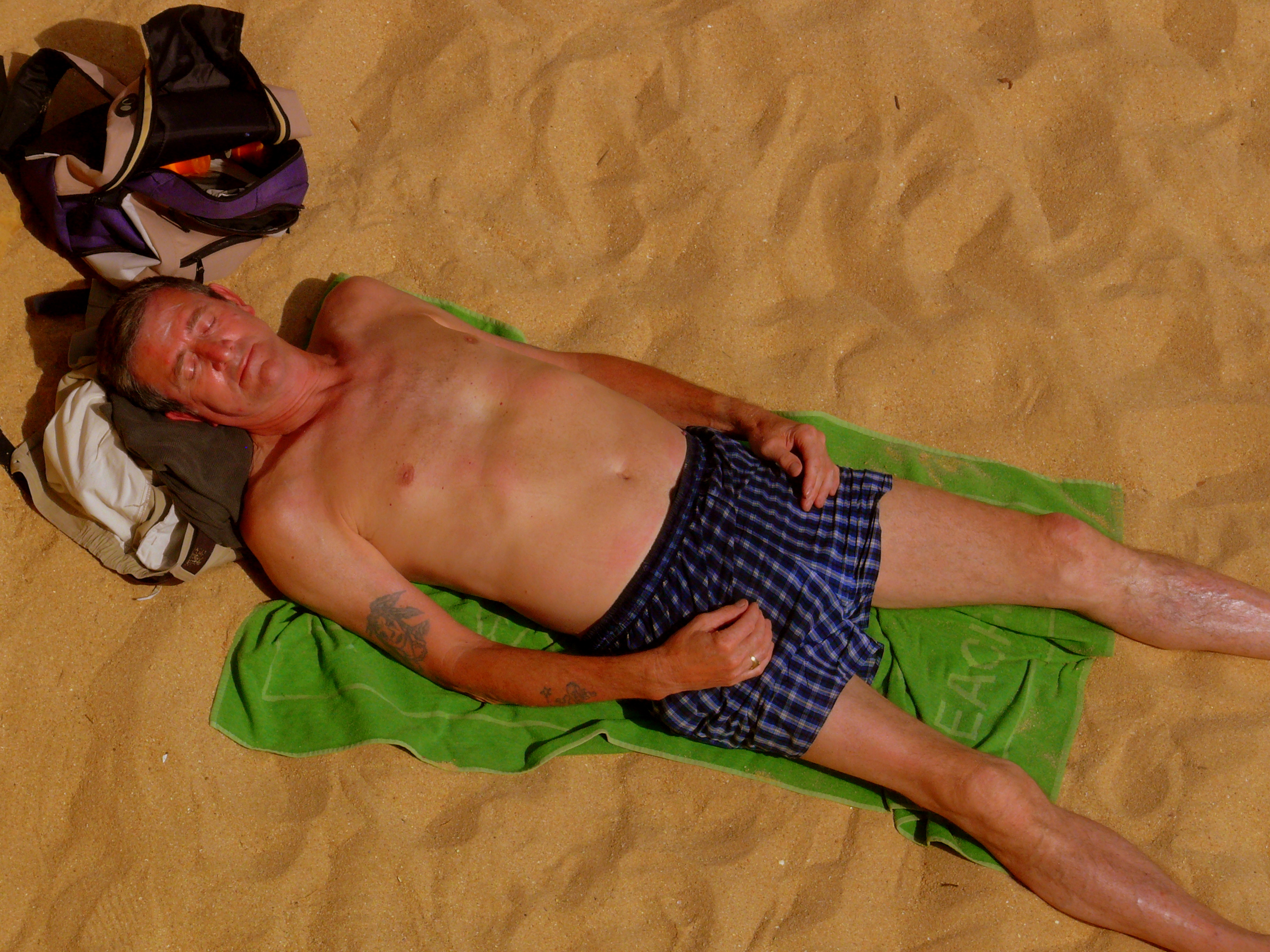An overhead shot taken at night with artificial reddish lighting captures a middle-aged man, seemingly in his 40s, lying on a light brown sandy beach. The man, with short dark hair, is positioned on a light green towel, which is approximately the size of his torso and marked with the text "EACH" near his knees. He appears to be sunbathing or resting, with his eyes closed and his face and arms markedly red, contrasting with the paler rest of his body. He is shirtless and wears blue plaid swim trunks. His head rests on his bunched-up pants, which feature a visible brown belt. To the left of his head in the image lies a backpack, purple and tan with black accents, containing indistinguishable items but showing some orange details. Notably, he has tattoos on his right arm, including an image resembling a Native American man with feathers in his hair, and wears a ring on his right hand.